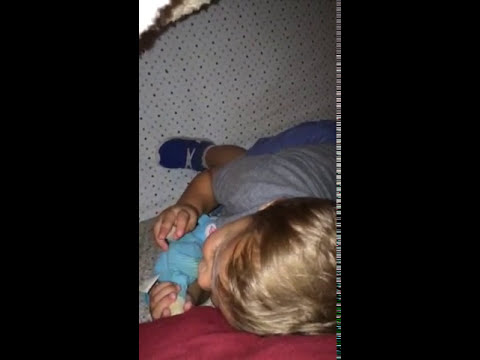A vertical top-view photo captures a toddler wearing a gray t-shirt, blue shorts, blue socks, and little blue shoes. The child has dirty blonde hair and a tan complexion. Resting their head against something red, possibly a blanket, a person's leg, or a chair, the toddler holds a light blue stuffed animal with discernible ears in both hands. The scene is set over a white polka dot blanket, and a tan-colored rug is visible in the background. The primary focus is on the child with the plush toy, providing a sense of warmth and comfort amidst the cozy, soft surroundings.